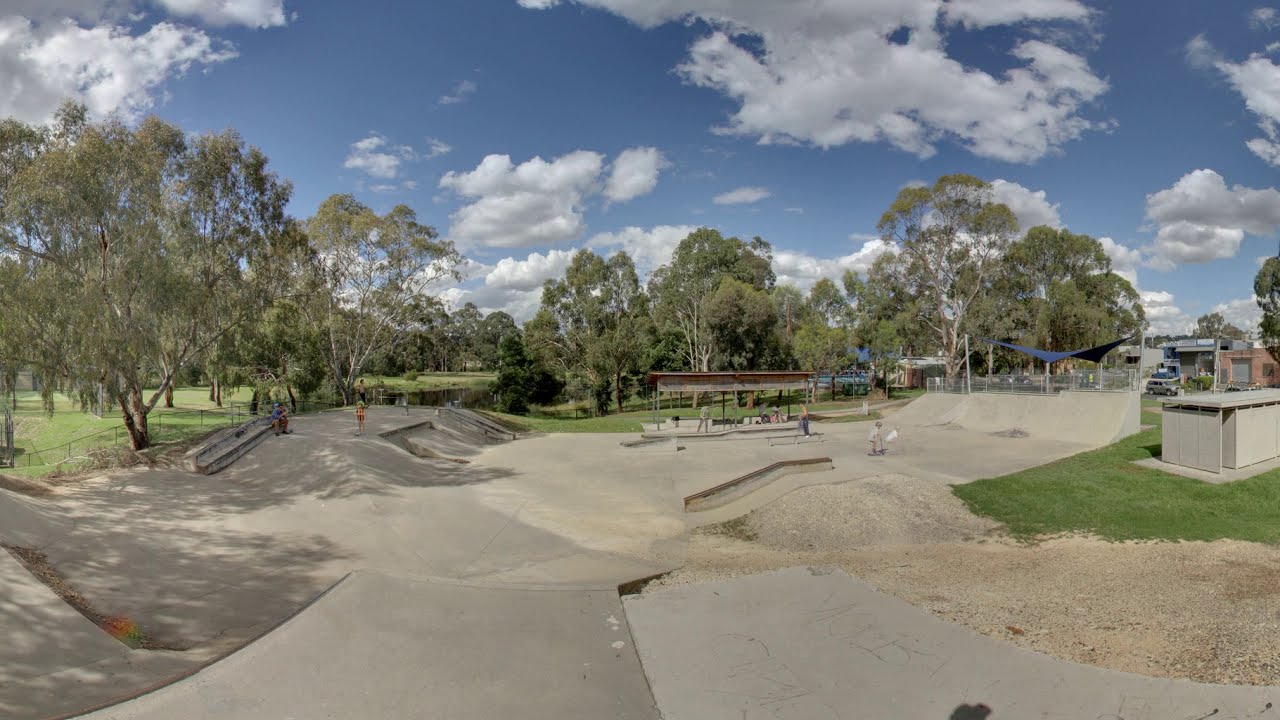The image illustrates a vibrant, outdoor recreational park area with a densely wooded backdrop. The central region features a network of sloping paths connecting motorboat pathways from the back left to the right. People are scattered throughout, with some walking, like the individual in a red shirt and shorts, and a couple seated on a stone bench on the left. Children can be seen riding scooters, utilizing the concrete ramps, and performing tricks on grindable walls. Adjacent to this, there are white stone benches for onlookers.

On the right, the landscape rises slightly to a wave-shaped umbrella cover, under which some people are gathered. In the same vicinity, there's a parked car against a red building with bluish windows. The background boasts a dense array of green, bushy trees, some thinner, allowing glimpses through the foliage. A chain-link fence encloses the park, beyond which lies lush green grass and tall trees. The sky above is a bright blue with fluffy white clouds. Additionally, another structure, described as a brown shed, sits centrally against the backdrop of greenery where more people congregate. This park area exudes a lively, community-focused atmosphere with ample open space and recreational facilities.